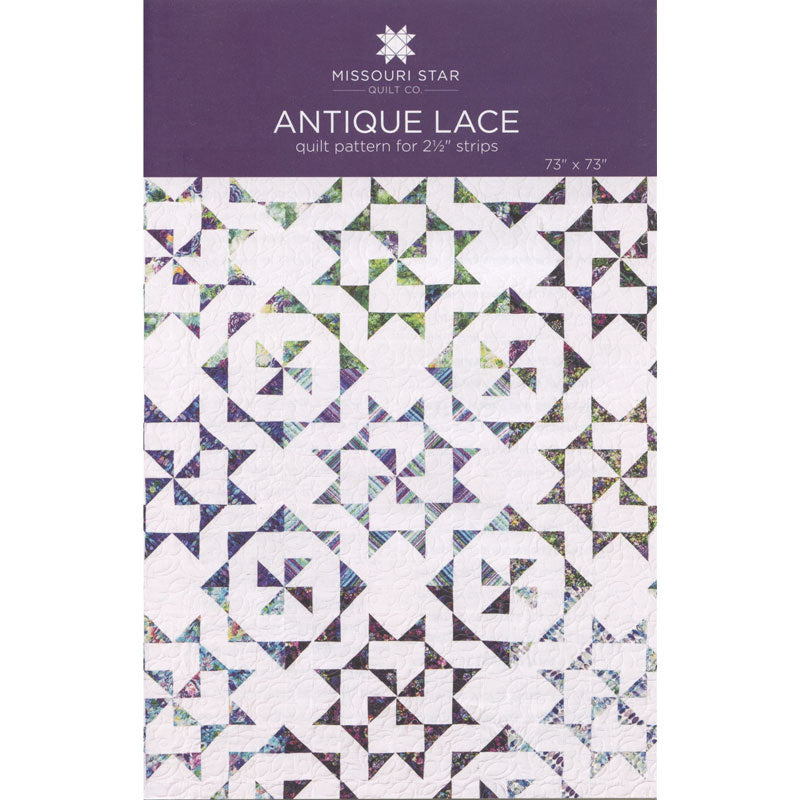"This is a poster advertising the Missouri Star Quilt Company featuring their 'Antique Lace Quilt Pattern.' At the top, there is a distinctive eight-pointed white star logo on a blue background, followed by the text in large white capital letters: 'Antique Lace Quilt Pattern for 2 1/2" Strips,' with dimensions '73" x 73" ' displayed in the bottom right corner. The main image showcases the quilt pattern itself, characterized by octagonal shapes resembling eight-sided stars or snowflakes, each adorned with a central motif of four fan-like petals. The intricate white lattice foreground contrasts beautifully with the vibrant green, purple, and blue hues of the background, creating a visually stunning and detailed design. It highlights both the pattern’s elegance and the rich colors that make it a standout quilting project."